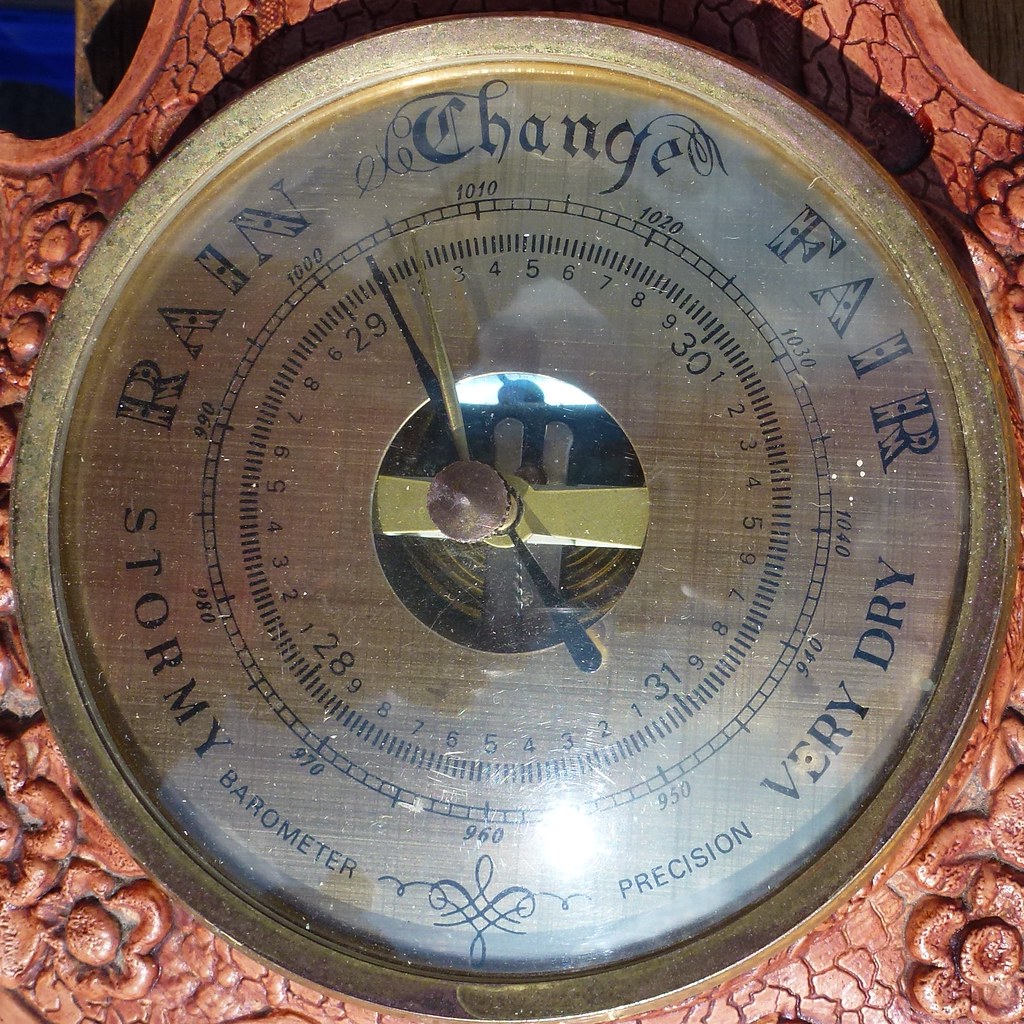This close-up photo captures an antique barometer embedded in what appears to be a carved wooden surface. The circular dial is predominantly golden with a surrounding gold rim. The outer edge of the dial displays weather forecasts in black lettering—stormy at 8 o'clock, rain, change at the top, fair at 2 o'clock, and very dry at 4 o'clock. Below this, a secondary scale, marked from 940 to 1040, encircles the main numerical scale ranging from 28 to 31 with smaller intervals marked from 1 to 9. The barometer's face also includes elaborate flowery lines and inscriptions such as "barometer" and "precision." A shiny, reflective center reveals intricate clockwork mechanisms, with the needle currently pointing towards approximately 28. The image background subtly features a pink hue with flower patterns, enriching the vintage aesthetic of the barometer.